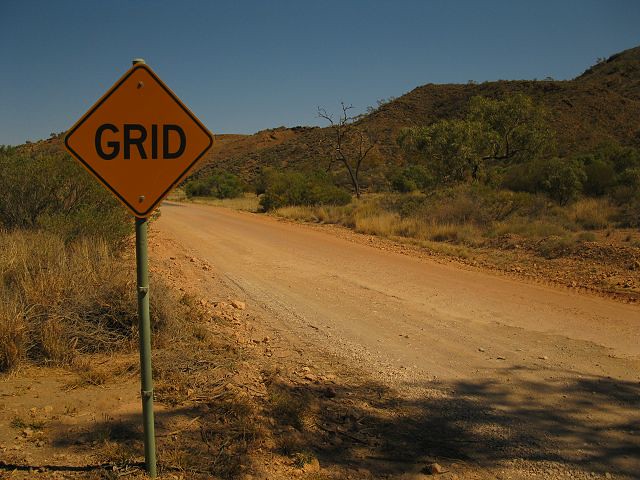This photograph captures a striking desert landscape featuring a tan-colored dirt road that snakes through the foreground. A green metal pole mounted with a yellow-gold sign bearing the black word "GRID" stands prominently on the left side of the frame. Scattered across the dry, patchy terrain are white-colored stones and a mix of brown, dark green, and light green grasses interspersed with various bushes. The scene is dotted with trees, some lush with green leaves and others bare, contributing to the area's rugged charm. In the background, gentle hills rise under a clear, blue daytime sky. Shadows of tree branches are visibly cast upon the dirt road, adding an intricate play of light and shadow to the composition.